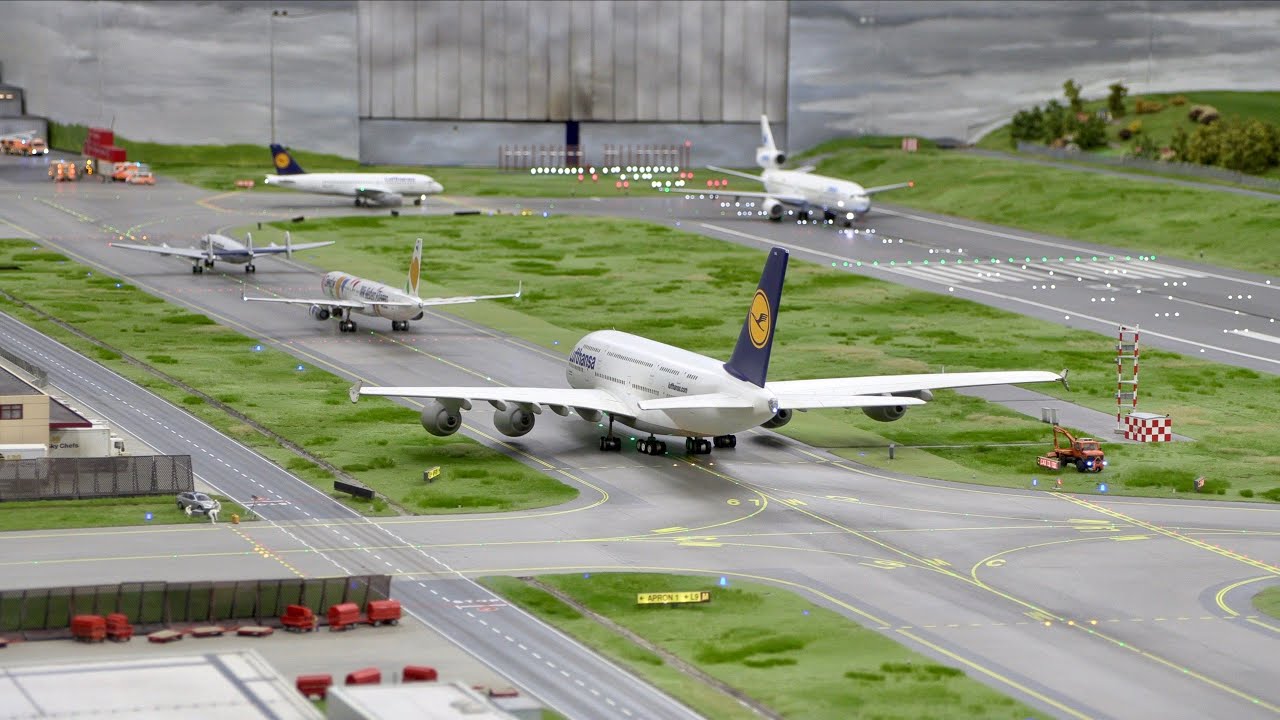This detailed image depicts a meticulously constructed model airport scene, showcasing five model airplanes lined up on the runways, ready for takeoff. Dominating the foreground, a Lufthansa plane stands out with its giant blue wing and the Lufthansa branding prominently displayed along its fuselage. Three additional planes can be seen on the left-hand runway, while another larger Lufthansa plane is positioned further ahead. The far-right runway features one more plane, all of which are stationary on airways encircled by green patches of grass. The intricate diorama includes numerous details such as green lights along the runways, tiny model vehicles, and scale-model buildings. Red containers are placed next to one of the buildings, and there are small signs dotting the scene. The backdrop reveals an overcast sky blending with an indistinct airport structure, complemented by green trees and faint glimpses of big trucks and car headlights, suggesting a bustling but miniature airport setting.